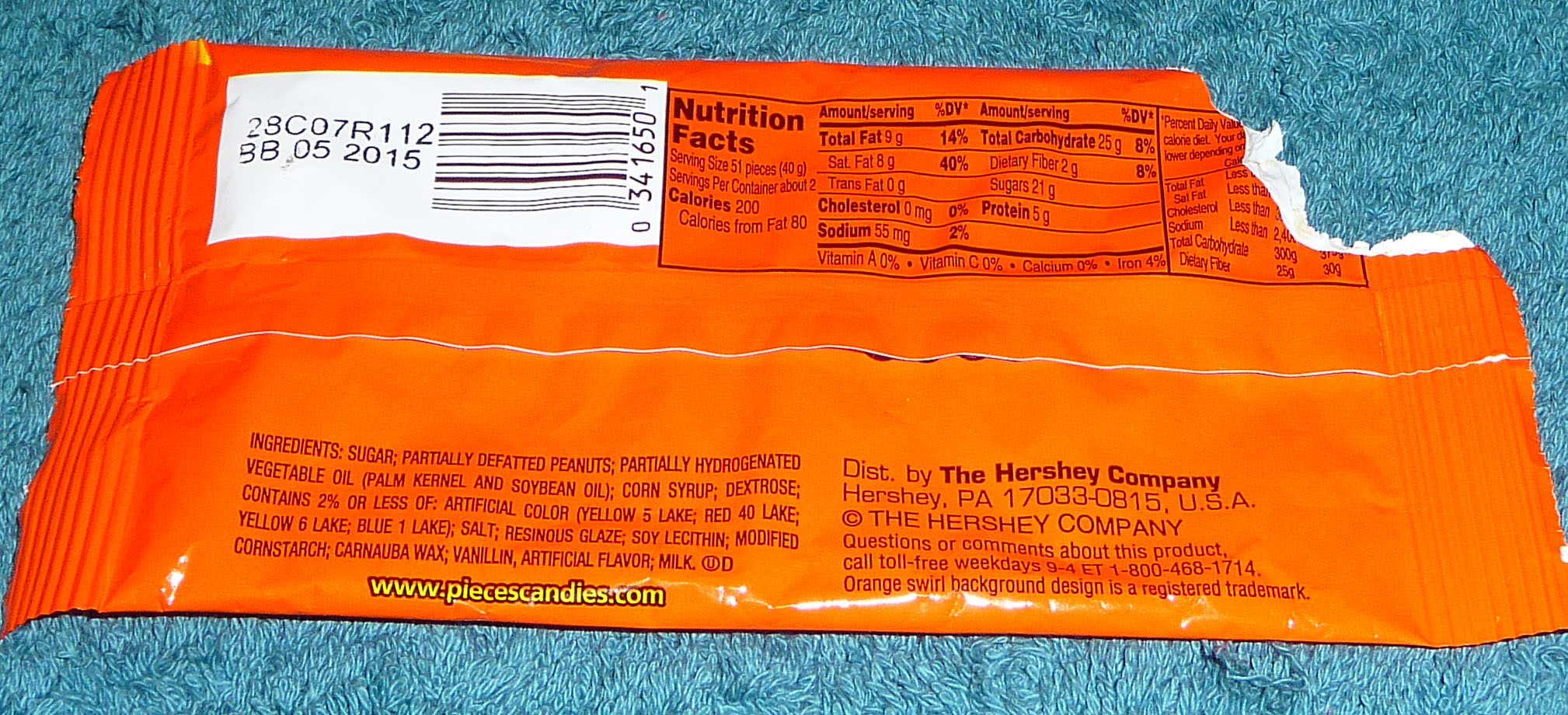A close-up image of an orange Reese's Pieces candy wrapper is laying on a teal-colored carpet, which, upon closer inspection, appears to be a blue towel based on the texture of the loops. The wrapper displays detailed nutritional information and ingredients. The package is slightly ripped on the right side, evidencing where it was opened. A white box on the left contains a UPC code (03416501) and a best before date of 05/2015, with the code 28C07R112. The nutrition facts on the right state that a serving size is 51 pieces, with about two servings per container. Each serving contains 200 calories, with 80 calories from fat. Additionally, each serving has 9 grams of total fat (14% of the daily value), including 8 grams of saturated fat (40% of the daily value), 0 grams of trans fat, 0 milligrams of cholesterol, 55 milligrams of sodium, 25 grams of carbohydrates, including 2 grams of dietary fiber and 21 grams of sugars, and 5 grams of protein. The wrapper also lists a lengthy ingredient list that includes sugar, partially defatted peanuts, partially hydrogenated vegetable oil (palm kernel and soybean oil), corn syrup, dextrose, less than 2% of artificial colors (Yellow 5 Lake, Red 40 Lake, Yellow 6 Lake, Blue 1 Lake), salt, resinous glaze, soy lecithin, modified corn starch, carnauba wax, vanillin (an artificial flavor), and milk. At the bottom, it states the distributor as the Hershey Company, Hershey, Pennsylvania, 17033-0815, USA, with a web address of www.piecescandies.com.